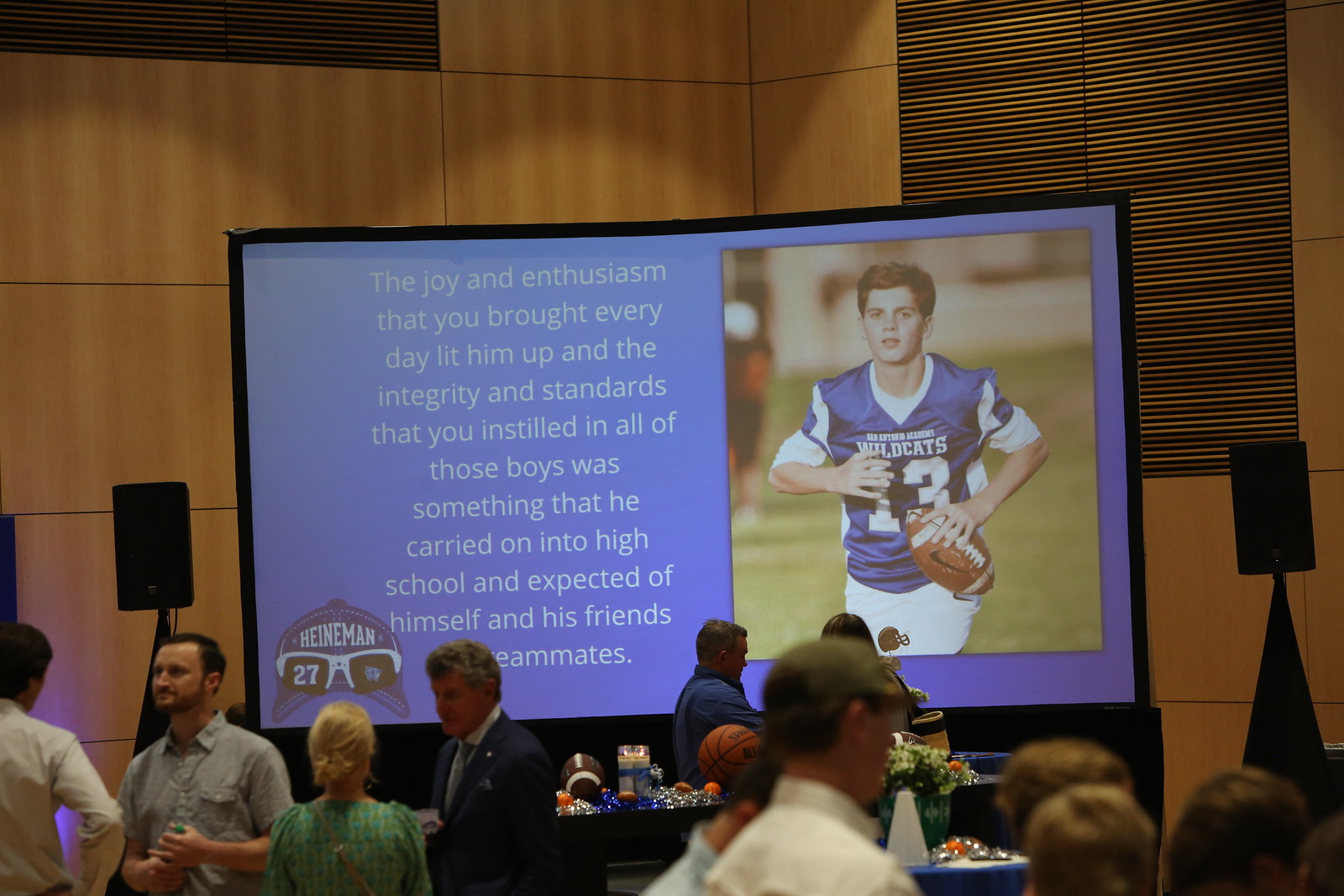The image captures a large meeting space, potentially an auditorium or banquet hall, with wood-paneled walls. At the center of the photo is a prominent projector screen displaying a young boy in a football uniform, labeled "Wildcats 13," holding a football in his left hand. To the left of the boy's image, white text on a blue background reads: "The joy and enthusiasm that you brought every day lit him up, and the integrity and standards that you instilled in all of those boys was something that he carried on into high school and expected of himself and his friends and teammates." Below the text, a blue illustration of a baseball cap with the word "Heinemann" and glasses perched on the brim, featuring the number 27 on one lens, is visible. In front of the screen, a table exhibits various items, including a football and a basketball. Numerous attendees, perhaps alumni, staff, and teachers, stand around the room engaged in conversation, emphasizing a lively and commemorative atmosphere.